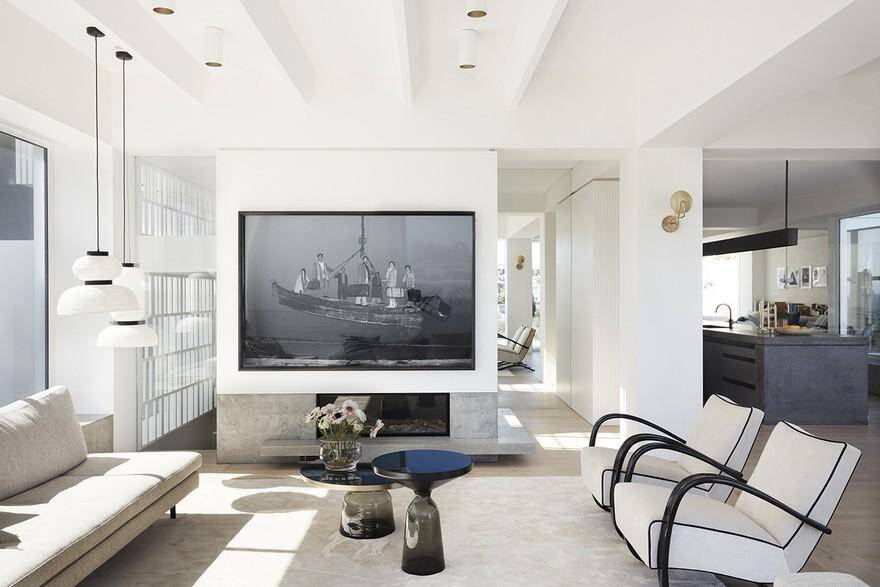This photograph captures the interior of a beautifully designed, monochromatic home with a modern aesthetic. The focal point in the center is a large TV set into the wall, which appears to show people on a boat. Below the TV is a sleek, modern fireplace. In front of this setup are two black and white armchairs facing left and a low white couch facing right, creating an inviting seating arrangement. Between the chairs are circular glass tables, one holding a clear vase with white flowers. A white rug anchors this seating area, complemented by two dark, likely black marble, side tables.

The walls are predominantly white, enhancing the room's clean and modern look. A large window on the left floods the space with natural light. Hanging from the ceiling are modern light fixtures with white lampshades, adding to the bright and airy feel. In the background, we get a glimpse of the kitchen, which features dark gray cabinetry and a concrete-looking island with a hook-shaped faucet. Above the kitchen area hangs a long rectangular light fixture. 

Notable elements include hints of gold, such as a sconce on the wall and recessed can lights, which add a touch of warmth and sophistication. A mirror strategically placed in the background creates an illusion of a larger space. The overall design reflects a meticulously styled, modern interior, likely staged for the photograph.